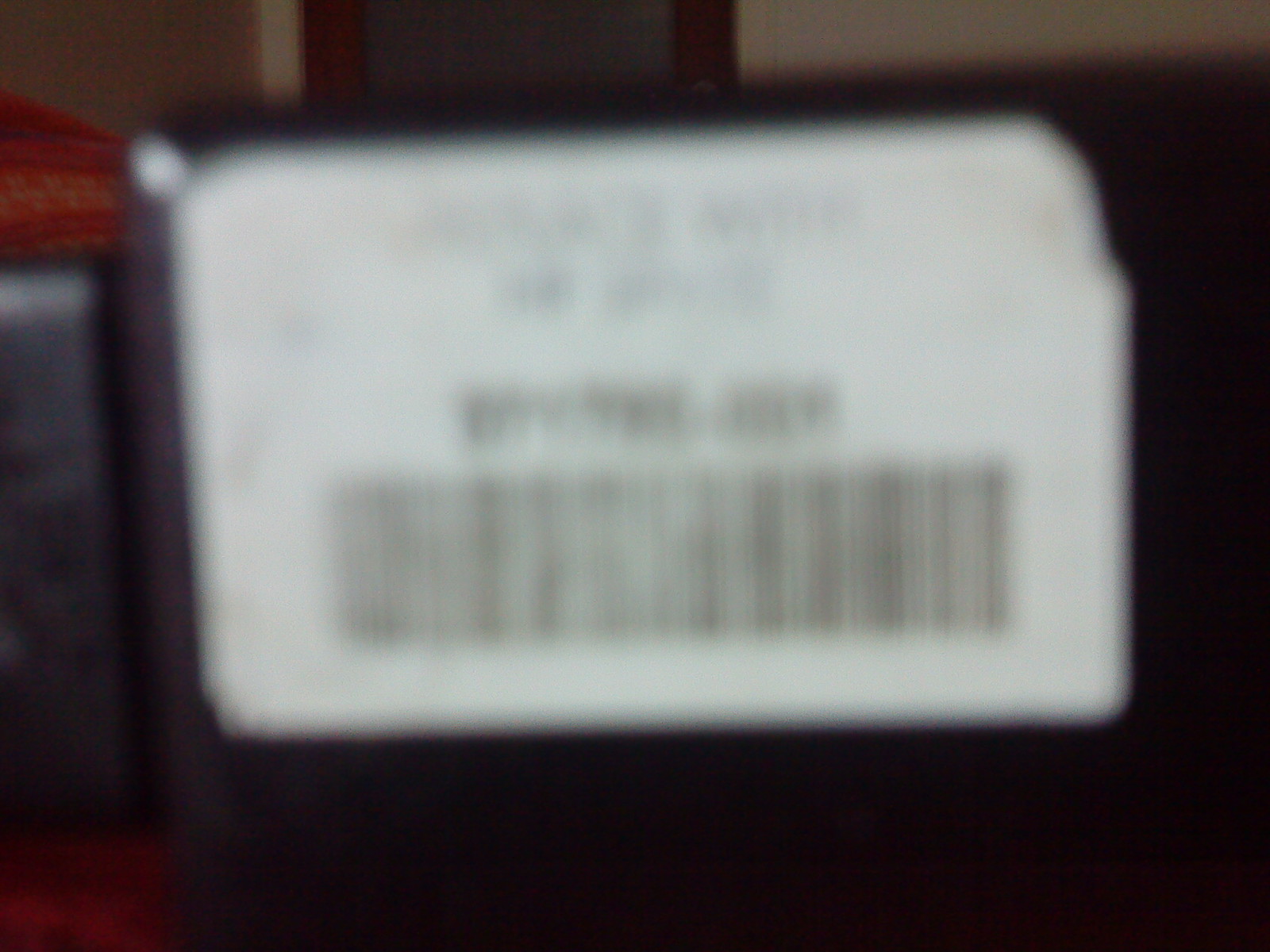A blurry image depicts a barcode printed on a white sticker, partially obscured by the blur. The sticker is affixed to a black, plastic object that has a shiny corner and appears very dark in the bottom right. Above the barcode, illegible text in both lighter and darker fonts is present, but the blurriness makes it difficult to discern any details. The black object seems to be connected to another item on the left, with a visible plug. In the background, there is a doorway with white walls and a brown door that features a glass panel in the middle. An indistinct orange object can also be seen on the left side of the frame.